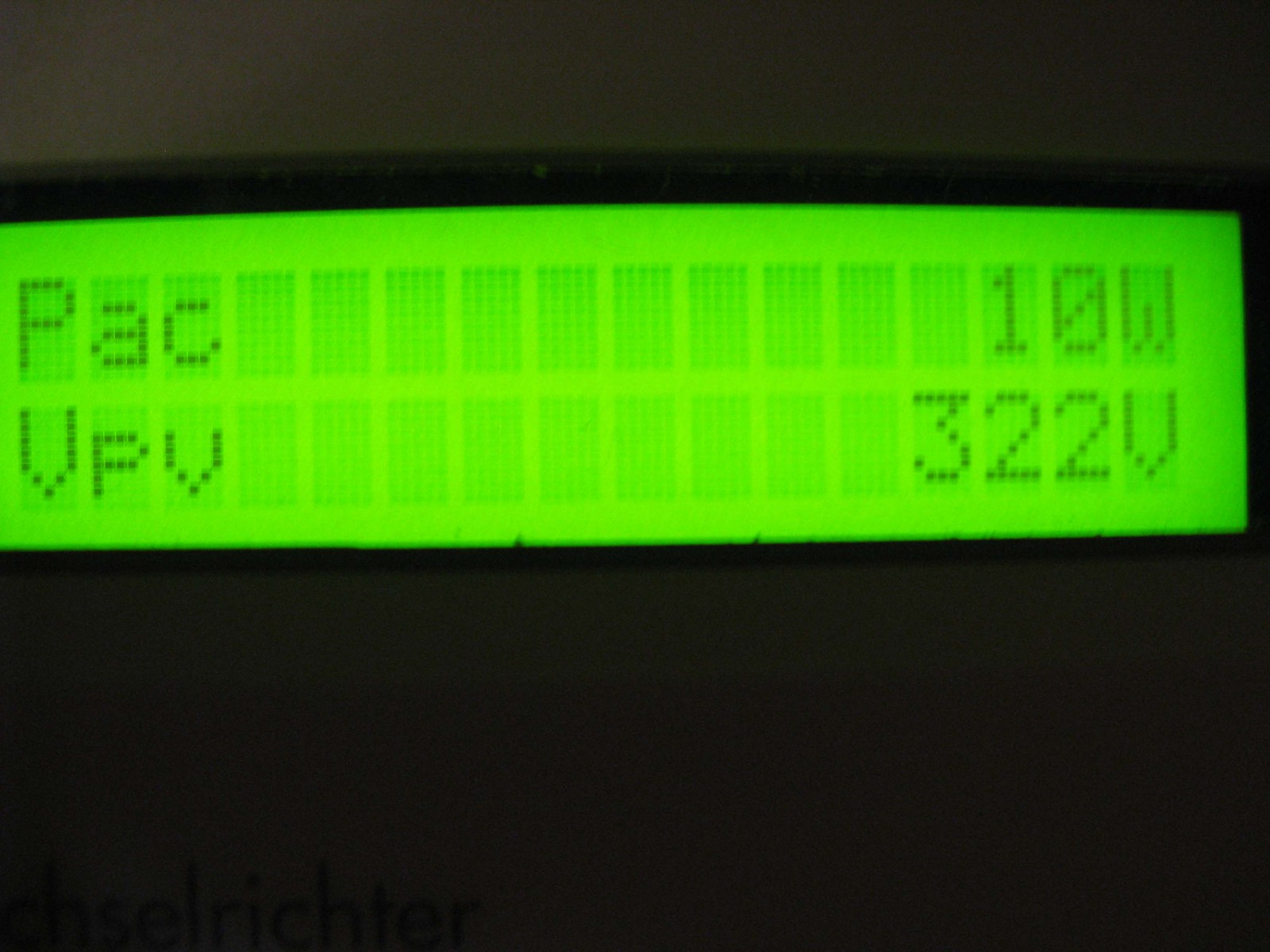The image depicts a long, thin rectangular electronic screen set against a completely black background. The screen itself emits a neon yellowish-green hue, reminiscent of an older digital display. It features two distinct rows of text comprised of letters and numbers. On the top row, from left to right, it reads "Pac" followed by "10W." The second row displays "VPV" on the left and "322V" on the right. The text appears within faint, almost burnt-in rectangles formed by tiny squares, giving the display an aged or vintage look.